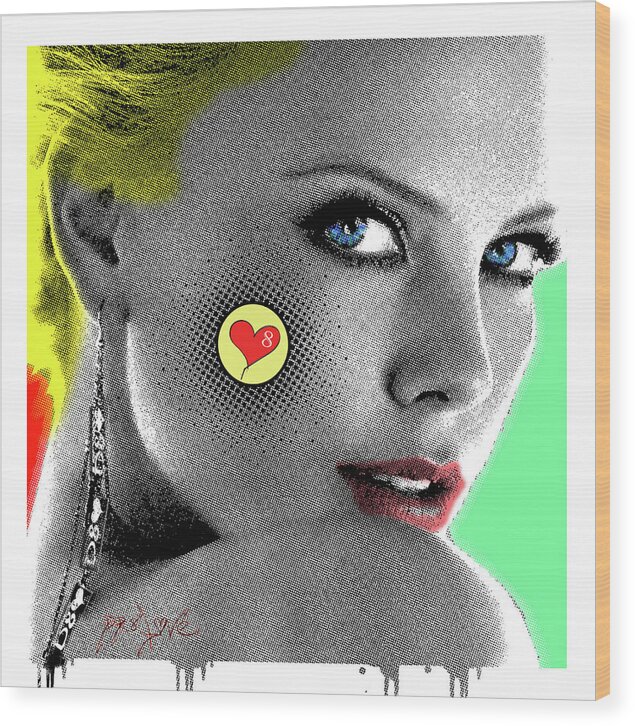This digital artwork, reminiscent of Andy Warhol's iconic Marilyn Monroe series, features a woman with fair gray and white skin tones that sharply contrast with her vibrant features. Her striking blue eyes peer over her shoulder directly at the viewer, framed by dark eyelashes. She sports bold red lipstick that stands out against her monochromatic complexion. Her hair is dyed an electric shade of yellow, bordering on a neon greenish hue.

Adorning her left ear is an extravagant silver earring that dangles down to her shoulder. A distinctive feature on her cheek is a pixelated design with a black outline; within this, a yellow circle surrounds a red heart, which itself encases a white number 8. The woman's shoulder has red script that appears to drip paint downwards, blending into the white border that encases the entire image. The vivid background transitions from a green adjacent to her face to a strip of red along her neck. The overall color palette includes shades of gray, yellow, red, green, and blue, creating a dynamic and visually arresting composition.